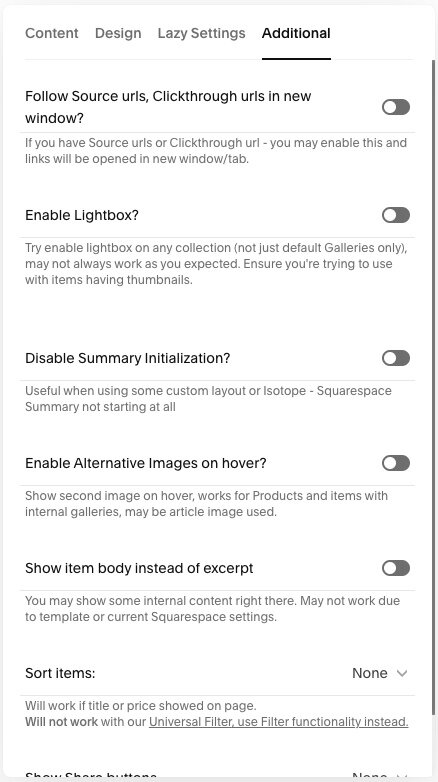This image is a screenshot taken from a cell phone displaying a settings menu. The background is predominantly white with gray accents, and features several toggle switches for different settings. On the right side of the screen, there are sliders that allow the user to toggle features on or off; the state of these sliders reflects if the toggle ball is positioned to the left (off) or right (on).

At the top of the screen, there is a navigation menu with the sections labeled "Content," "Design," "Lazy Settings," and "Additional," with "Additional" appearing slightly bold and underlined, indicating that it is the current active section.

Below this navigation section, a list of settings options is displayed:
1. "Follow Source URLs, Click Through URLs in New Window" - toggled off.
2. "Enable Lightbox" - toggled off.
3. "Disable Summary Initialization" - toggled off.
4. "Enable Alternate Images on Hover" - toggled off.
5. "Show Item Body Instead of Excerpt" - toggled off.
6. "Sort Items" - set to "None."

Each setting option includes a descriptive label alongside its respective toggle switch, illustrating which features are currently enabled or disabled.